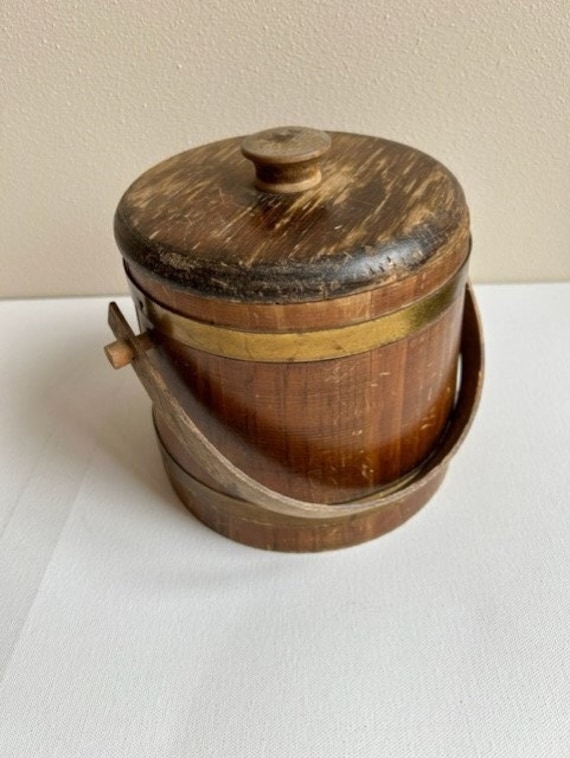The image features a close-up photograph of a small, old-fashioned wooden bucket with a lid. The bucket, which sits on a white surface, possibly a table, is positioned against a light beige, textured wall. The wooden body of the bucket shows signs of wear and is stained in medium brown hues. The lid has a darker brown knob-like handle, giving it the appearance of a drawer pull. The bucket is reinforced with two bronze or gold-colored metal rings, one around the top rim and another at the bottom. A single wooden peg on the side of the bucket secures a long, rounded handle, which rests against the body of the bucket when not in use. The overall close-up perspective of the photo isolates the bucket as the central focus, emphasizing its rustic and functional design.